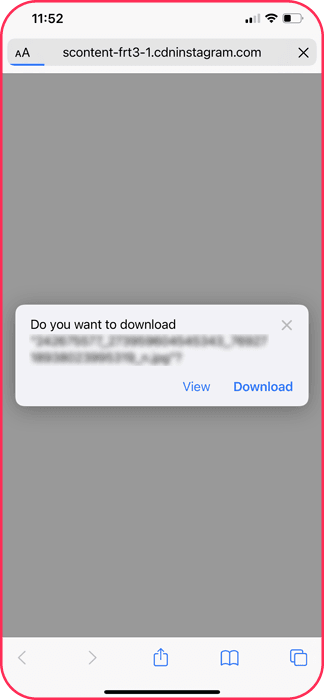The image depicts a screenshot taken from an iPhone, displaying a Safari browser page. The website URL visible at the top is "scontent-frt3-1.cdninstagram.com," indicating the user is trying to interact with content hosted on Instagram's CDN. There's a prominent red outline around the phone's interface. In the center of the screen, a pop-up dialog asks, "Do you want to download?" with options for "View" or "Download," though the exact file is obscured by a gray placeholder image.

The time, shown at the upper left, reads 11:52, while the upper right corner displays the Wi-Fi signal and battery level indicators. Standard Safari navigation buttons are present at the lower part of the screen, allowing users to go back, forward, or open multiple tabs, among other functions. A black bar at the bottom suggests the presence of a virtual home button, consistent with newer iPhone models. Overall, the screenshot captures a moment where the user is prompted to download content from Instagram via Safari on their iPhone, though the specific content remains undetermined due to blurring.